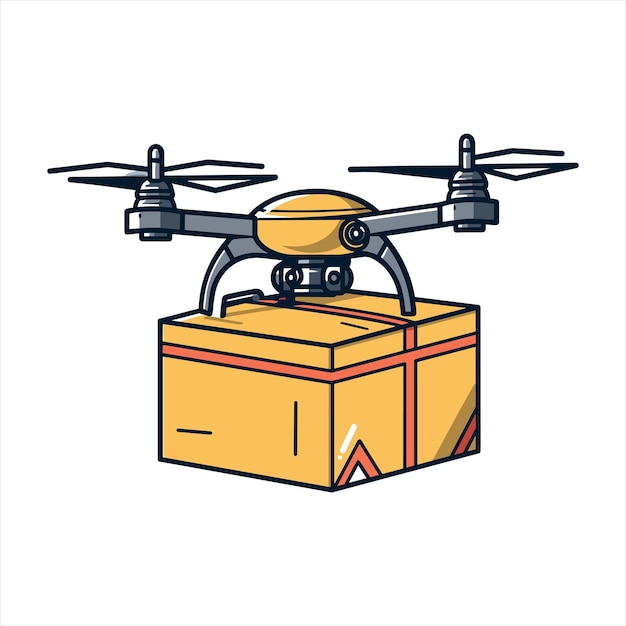This image is a detailed illustration of a silver drone with a yellow body, equipped with two propellers and three legs, which are attached to a medium-sized box. The box is yellowish-tan and features red tape arranged in a cross pattern on the right side, with additional triangular shapes of tape on the bottom corners. The drone’s central body, matching the yellow of the package, is secured with visible metal screws and appears to have cameras. The box, resembling a present, is orange-yellow with white accents. The background of the image is completely blank, emphasizing the drone and package.